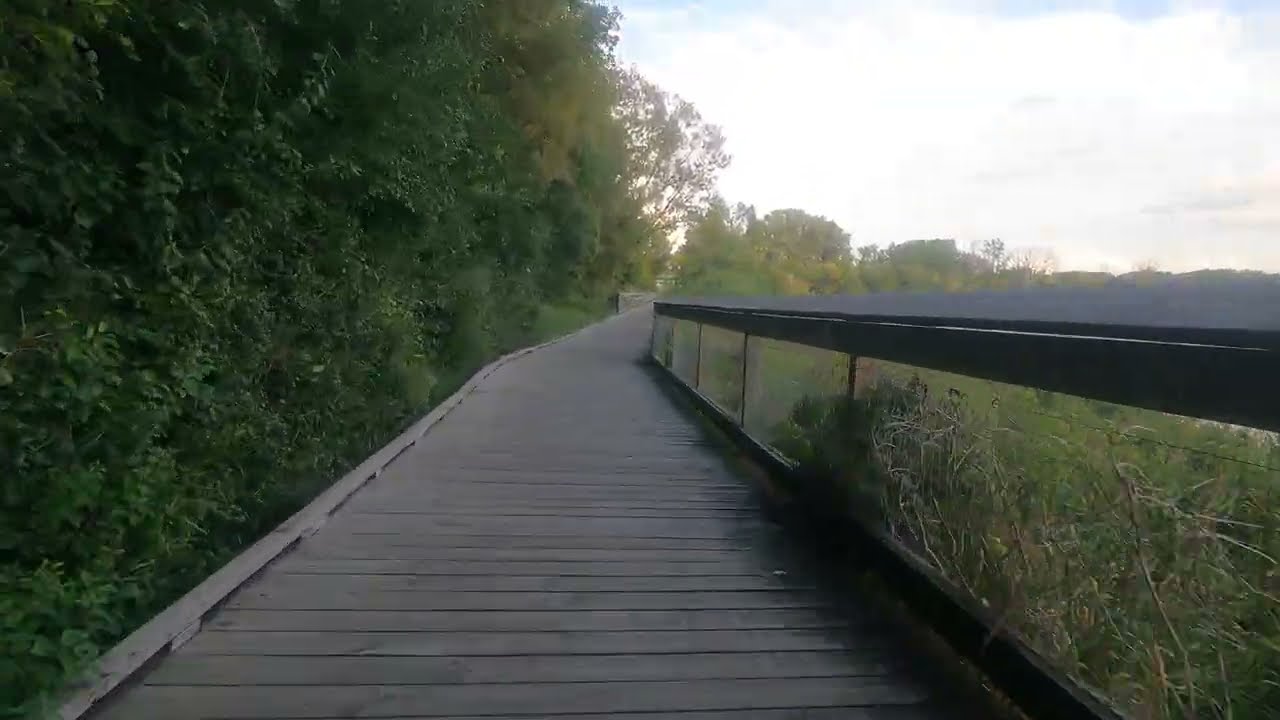The image captures a serene wooden walkway meandering through a lush natural area, viewed from the perspective of someone walking along the path. On the left side, a dense cluster of tall trees fills the scene, with their greenery creating a wall of foliage, while the right side is lined with smaller plants and a wooden railing. The walkway, resembling a wooden bridge, is made of two-by-four planks laid out consecutively, leading from the bottom center of the image up to the middle. In the upper right corner, the sky is visible with patches of light blue and scattered clouds, and there is a hint of sunlight breaking through from the left. The color palette includes various shades of green from the trees and plants, as well as hues of tan, brown, gray, and touches of yellow, orange, white, and light blue. There are no people or text in the photo, emphasizing the tranquility of the midday outdoor setting.